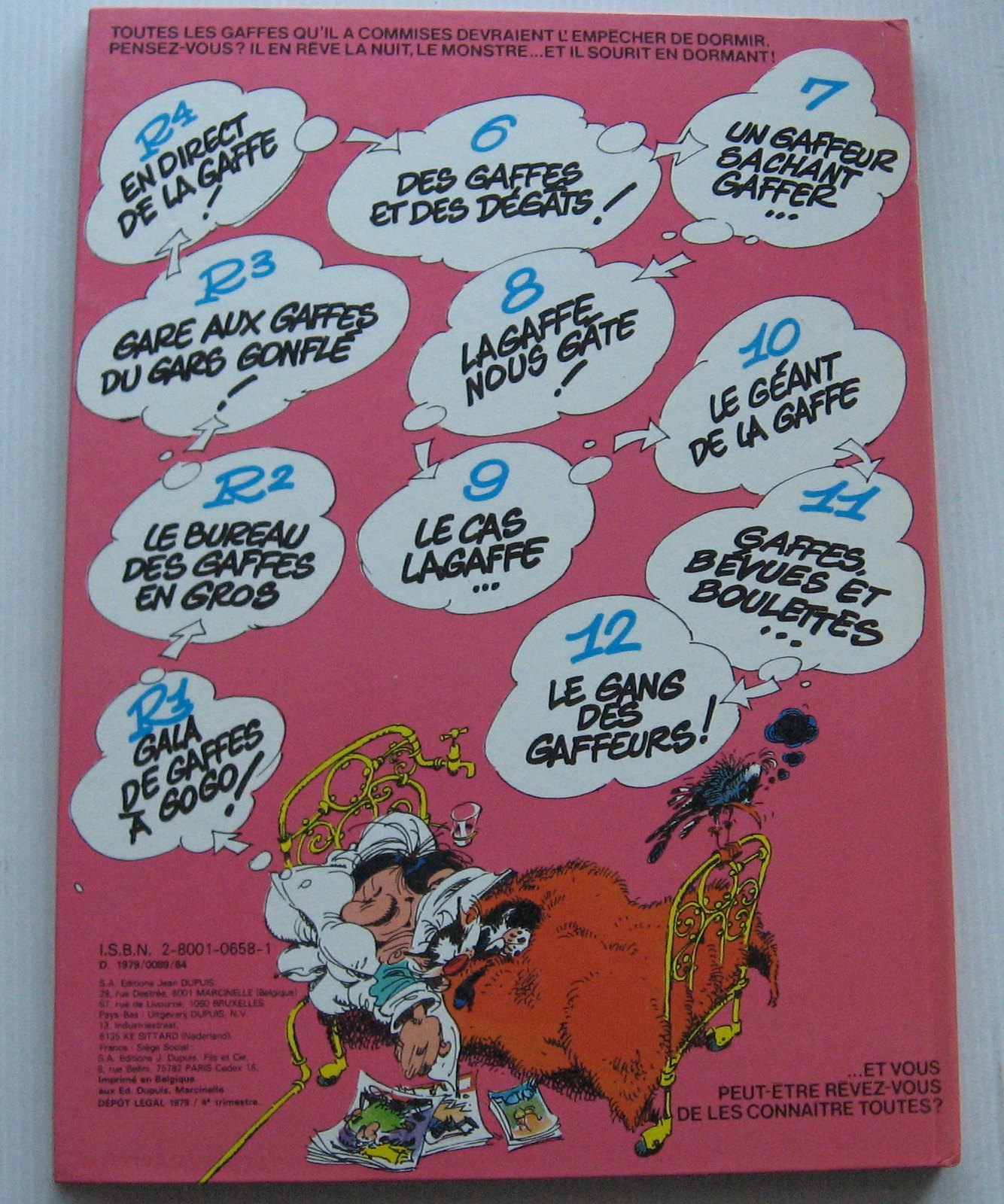The image depicts the packaging of an unknown item with a pink background, annotated mostly in French. It features a detailed cartoon of a man with dark hair and a large nose, sleeping in a gold-framed bed with a white pillow and a furry red blanket pulled up to his face. He is accompanied by a cat sleeping at the foot of the bed and a bird perched on the bed frame. The bed also has an unusual attachment of a tap with a receptacle below it.
 
On the floor beside the bed, there are several magazines. Above the sleeping man, about a dozen blue text bubbles with arrows connecting them display various French phrases and numbers, including sequences like R2, R3, and so forth. Additional French text is found along the top and bottom of the packaging, although the specific meanings of the phrases remain unclear. There's also an ISBN number located in the bottom left corner. The overall scene suggests the man is deep in sleep and possibly dreaming, as indicated by the interconnected thought bubbles above him.